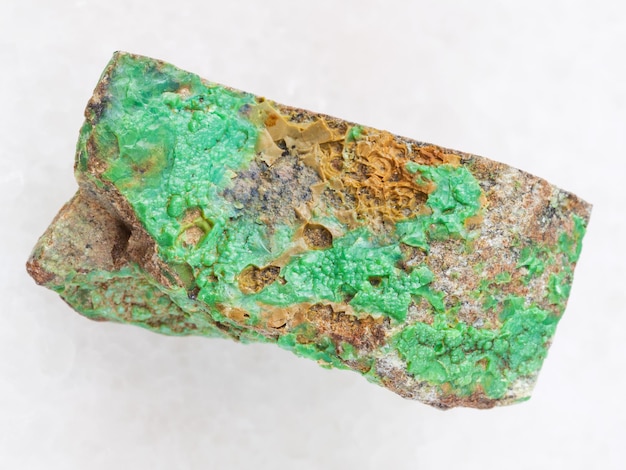The image depicts a rustic piece of bread, possibly ciabatta or focaccia, situated on a plain gray-white background, reminiscent of a science book photograph. The bread displays significant mold growth, with a vibrant, smooth, and bubbly green substance covering a large portion of its surface, creating an almost gel-like appearance. Beneath the mold, a scant smear of peanut butter is visible, along with a hint of another dark-colored substance, suggesting an attempt to make a peanut butter and jelly sandwich. The bread, which appears to have been split and one half placed atop the other, shows signs of having been left out for several days, leading to a textured, puckered effect from the mold's spread.